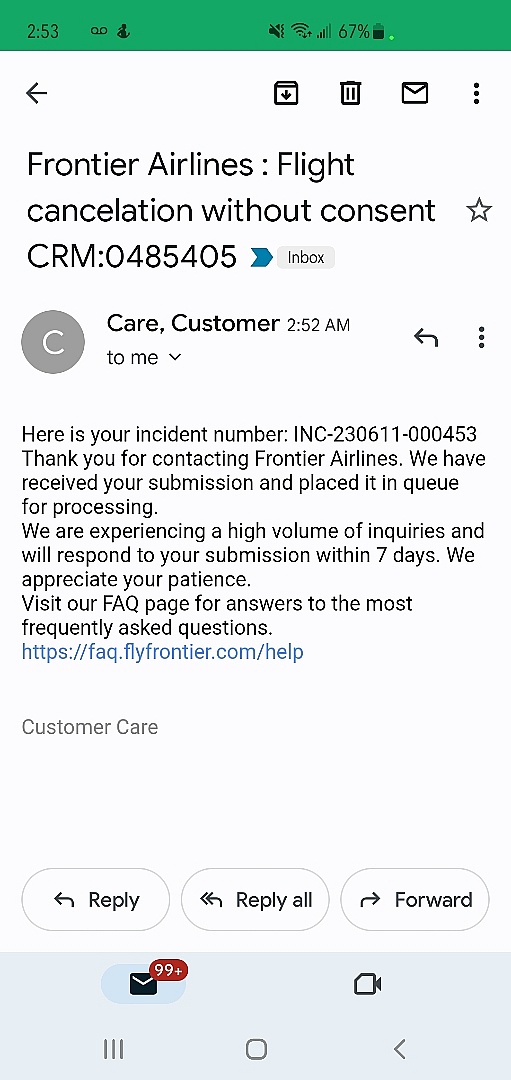Screenshot of an email displayed on a cell phone screen, featuring a message from Frontier Airlines. At the top of the image, the cell phone status bar is visible, indicating the device's signal strength, battery life, and other standard icons.

Beneath the status bar is an email notification in enlarged black font on a white background, with the subject line: "Frontier Airlines Flight Cancellations Without Consent. CRM 0485 405". The email is addressed from "Customer Care" to the recipient.

The body of the email contains an incident number "INC230611-000453" followed by the message: "Thank you for contacting Frontier Airlines. We have received your submission and placed it in queue for processing. We are experiencing a high volume of inquiries and will respond to your submission within 7 days. We appreciate your patience. Visit our page for answers to the most frequently asked questions: https://flyfrontier.com"